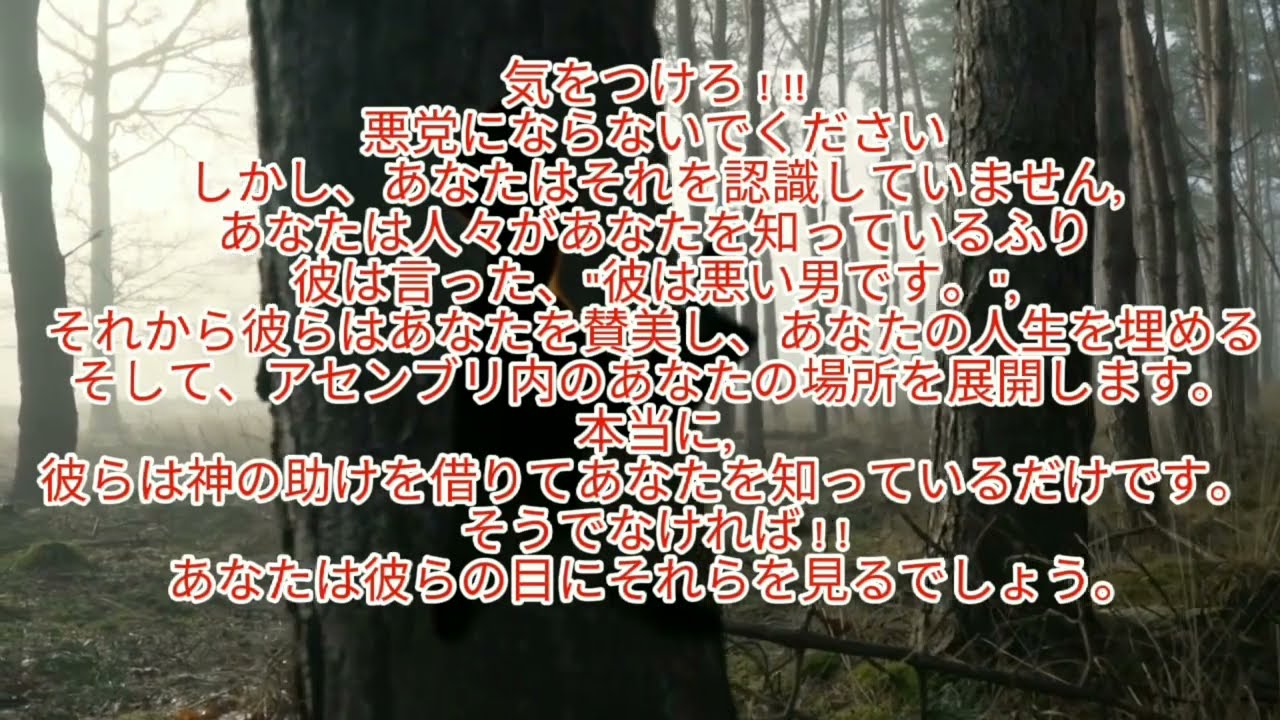The image captures an eerie, dense forest scene, likely taken at ground level near a river or stream. Foregrounded is a particularly thick brown tree trunk that dominates the left side of the photo, with another equally robust tree trunk situated further to the right. Scattered throughout the forest floor are dark brown dead branches, green moss, and brown leaves, contributing to the overall dark greenish-gray hue of the ground. In the background, thinner and scrawnier tree trunks fade into a hazy white fog, enhancing the image's spooky atmosphere. The sky overhead is completely gray, casting an eerie, dull glow over the entire scene. Superimposed across the center of the photo, in vibrant red bubble letters with white borders, are multiple rows of Asian characters, resembling the end credits of a television show. These characters are densely packed, nearly filling the middle of the image, adding to the surreal quality of the scene.